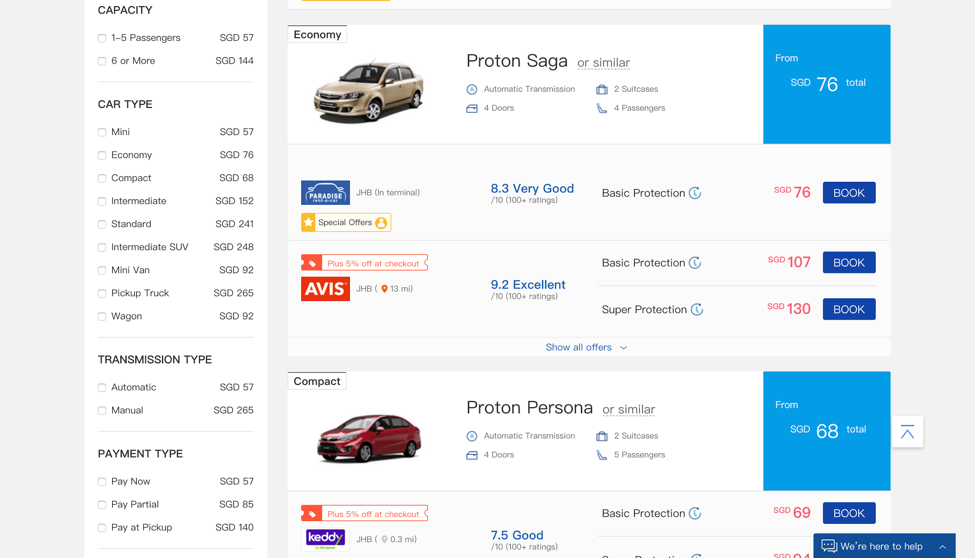The image depicts a detailed layout of a car rental booking website displayed on a computer screen. On the left side of the screen, there is a white menu bar divided into several sections:

1. **Capacity** at the top: Options include "one to five passenger car" and "six or more passenger car."
2. **Car Type**: The categories listed are mini, economy, compact, intermediate, standard, SUV, minivan, pickup truck, and wagon.
3. **Transmission Type**: Choices available are automatic and manual.
4. **Payment Type**: Options include "pay now," "pay partial," and "pay at pickup."

On the right side of the screen, an economy car option is shown with a small gray car image labeled as "Proton Saga or similar." There is a prominent blue square to the right that states "From $76 total." Below this, ratings and booking options are provided:

- **Paradise Rental**: 8.3/10 rating (Very Good). You can book this option for $76 by clicking a blue "Book" button.
- **Avis**: 9.2/10 rating (Excellent). The base rate is $107 with basic protection, and $130 with super protection, both of which can be booked by clicking a blue "Book" button.

Below this, the compact car option showcases a red car labeled "Proton Persona." The price starts "From $68 total." Additional details include:

- **Kennedy**: 7.5/10 rating (Good). The basic protection rate is $69, available for booking via a blue "Book Now" button. 

This comprehensive layout makes it easy to compare and book different car rental options based on type, transmission, payment preferences, and ratings.